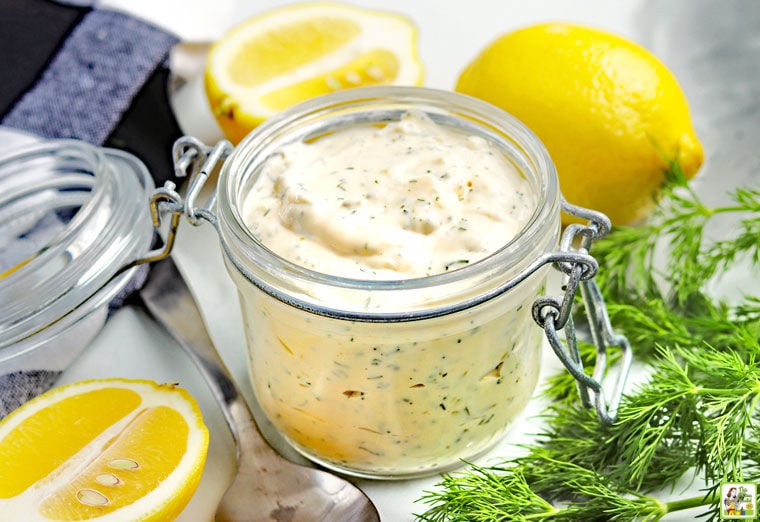This photograph captures a close-up, inviting kitchen scene centered around an open mason jar with a hinged lid, revealing a creamy, thick mixture that appears to be a homemade dip or spread, possibly aioli or cream cheese-based. The mixture is adorned with visible herbs like dill and possibly thyme or rosemary, enhancing the notion that it is freshly prepared. Surrounding the jar are complementary ingredients: a whole lemon, a halved lemon with three visible seeds in each half, and scattered sprigs of herbs. A spoon lies to the left of the jar, nestled between the lemon halves and ready for scooping the dip. The setting exudes a clean, holistic vibe, suggesting a healthy and appetizing option for a meal.